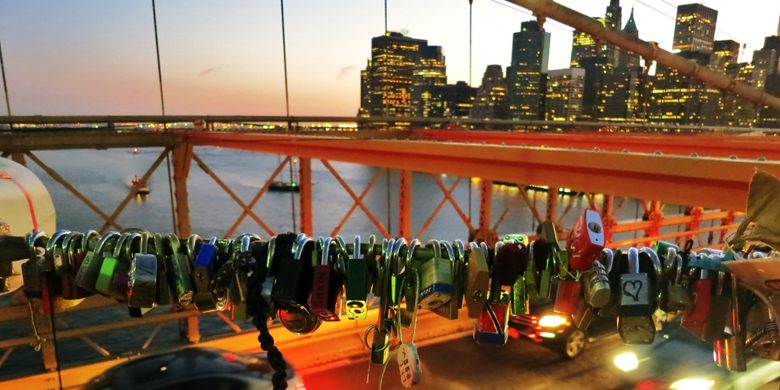This vibrant photograph captures an orange metallic suspension bridge adorned with a colorful array of interlocking padlocks in the foreground. Each padlock varies in shape, size, color, and type, with some displaying distinctive features like a Master brand label and heart engravings. The bridge spans over a body of water, with boats visible below. To the right, the background features a sprawling cityscape with illuminated skyscrapers, their lights casting a yellow glow at dusk or dawn. The sky is painted in soft hues of yellow-pink, indicating the sun has either just set or is about to rise, setting a serene, yet vibrant, scene over the tranquil water.